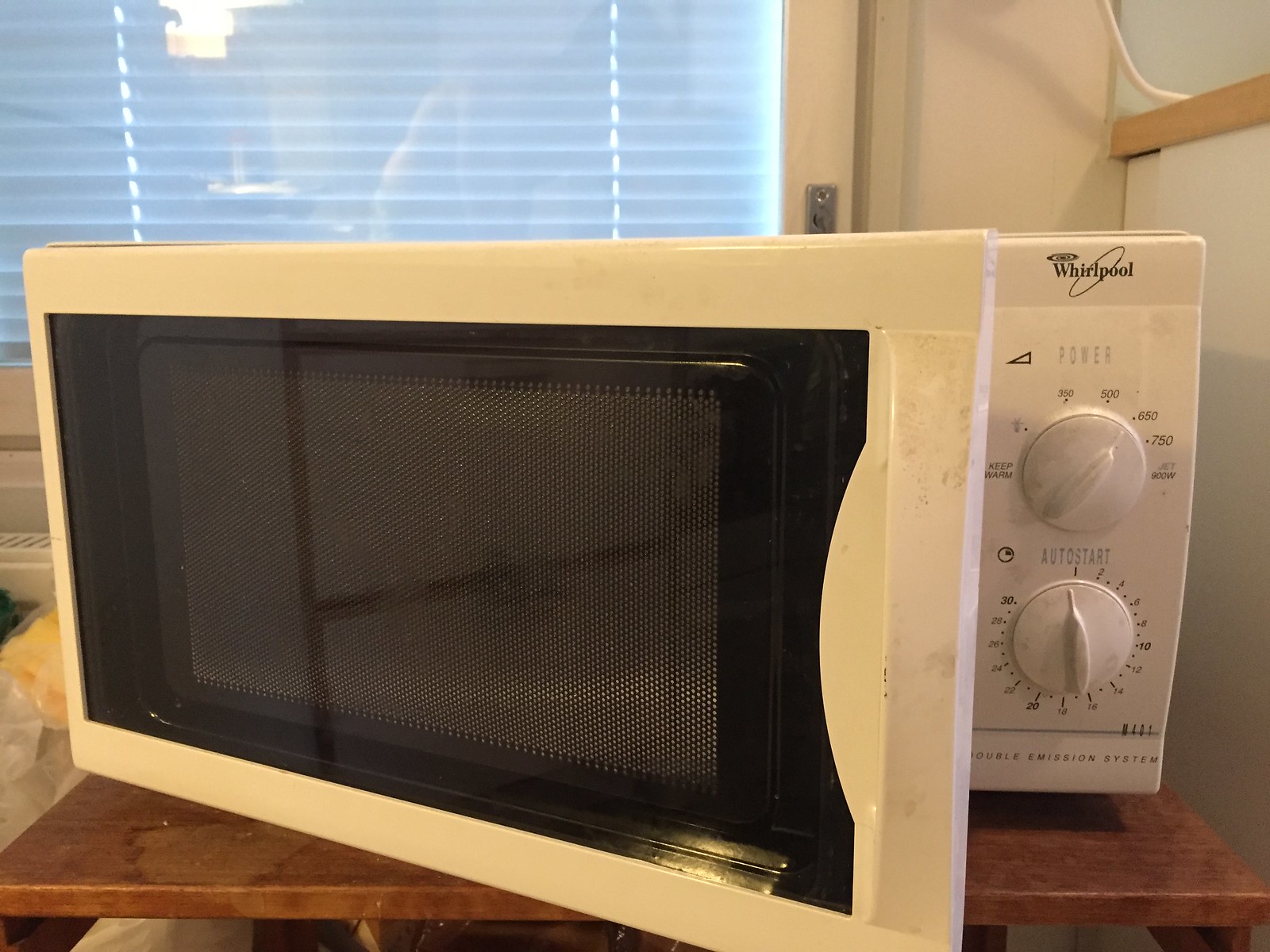This detailed photograph showcases a vintage ivory-colored Whirlpool microwave oven prominently positioned on a slightly stained, brown wooden table. The microwave's design features aged plastic dials on the right side, used for manual controls. The upper dial, labeled "POWER" in uppercase gray letters, provides various cooking intensities, including settings like "keep warm," "350," "500," "650," "750," and "jet." The lower dial, labeled "AUTO START," allows time adjustments in two-minute increments, ranging from 1 to 30 minutes and marked with intermediate dots for precision. Below these dials, the microwave boasts the "Double Emission System" inscription, hinting at its advanced heating technology for its time. The door of the microwave is slightly ajar, revealing the characteristic black, grid-patterned window designed to retain heat and allow visibility. This window is barely transparent but reveals a glimpse of a rotating plate inside. The microwave sits against a backdrop of a window fitted with white micro blinds, with a small portion of a white wall visible to the right. Additionally, a wire hangs subtly from the upper right corner, adding to the nostalgic feel of this quaint kitchen setup. The handle of the microwave shows some gray-black smudges, indicating frequent use and adding to the vintage charm of the scene.